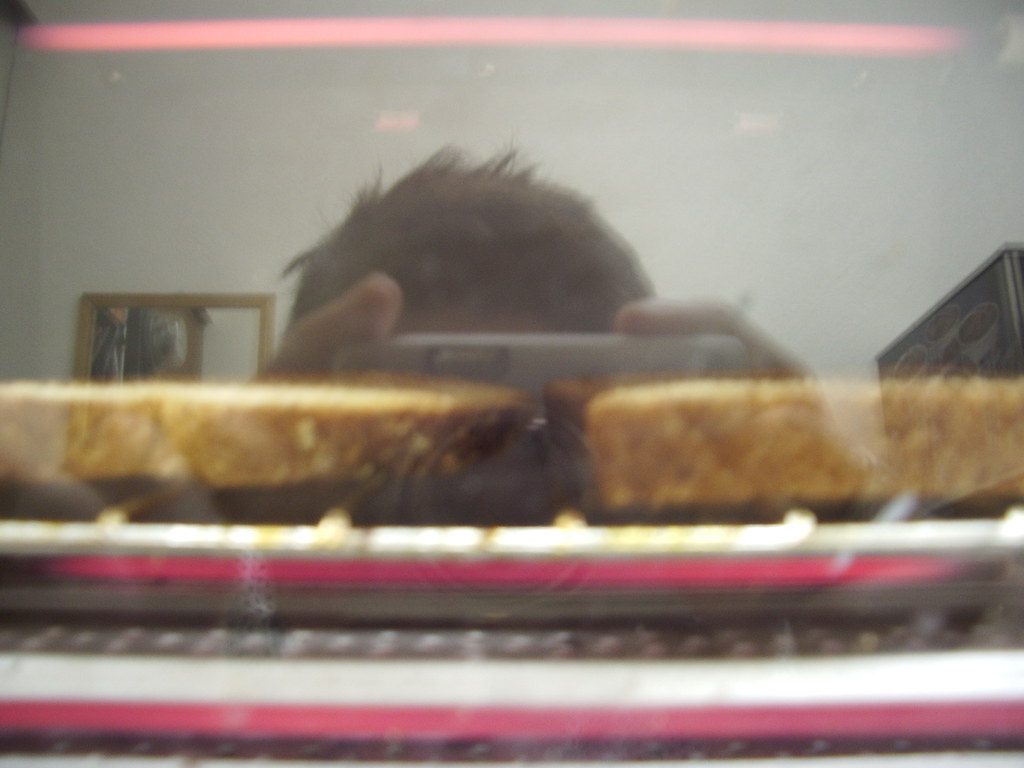This is a color photograph, slightly out of focus, likely taken through a glass surface. The reflection reveals the photographer, identifiable by their short brown hair, holding a camera phone or a silver camera with a large black lens, which they stabilize with both hands. Their unkept hair is faintly visible at the top of the frame. The main focus of the photo is a pair of food items, possibly cakes or pizzas, positioned on a tray or in an oven. Prominently, there are two horizontal white lines below these food items, followed by pink lines, all set against a grey background. Above, there's another horizontal pink line. To the left of the photographer's head, a picture frame or a mirror with a brown frame is visible. On the right side, the reflection displays another dark, square object. Overall, the scene is backdropped by a light blue sky and a black billboard.